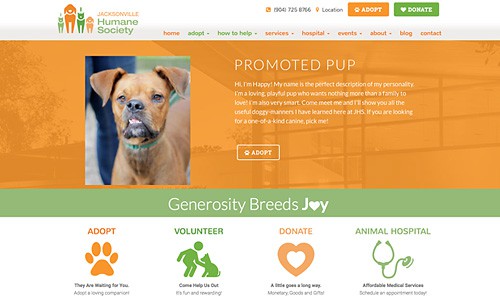The Jacksonville Humane Society's website prominently displays its branding with an appealing mix of colors and images. In the upper left corner, digital illustrations of dogs and cats catch the eye, with two orange and two green figures. The site's name is split, with "Jacksonville" in vibrant orange and "Humane Society" in lively green.

At the top, viewers can find crucial information, including a phone number and location. Quick-access buttons, "Adopt" in orange and "Donate" in green, invite user interaction. Further navigation options such as Home, Adopt, How to Help, Services, Hospital Events, About, Blog, and Contact ensure users can easily find what they're looking for.

Centrally featured is an adorable tan dog with floppy ears and a black nose, slightly open mouth, highlighting a playful yet serene expression. The dog, adorned with a green collar, is showcased as the "Promoted Pup," embodying a friendly and happy demeanor. The accompanying text warmly introduces him with, "Hi, I'm Happy. My name is the perfect match for my personality," followed by more details about him.

A prominently placed button encourages visitors to "Adopt Happy," and a green bar beneath declares "Generosity breeds joy," with the 'O' in "joy" rendered in a heart shape. At the bottom of the page, easy access options for "Adopt," "Volunteer," "Donate," and information about the "Animal Hospital" streamline user actions, fostering engagement with the Humane Society's mission.